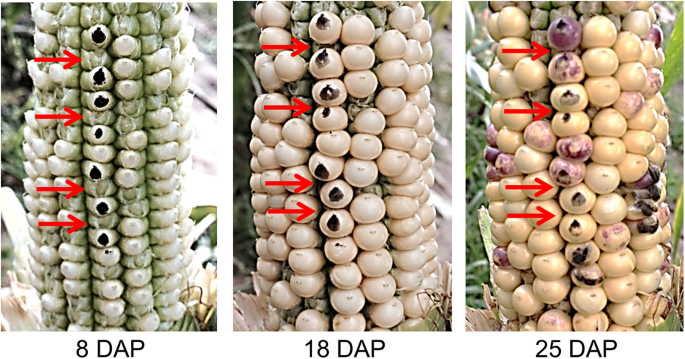This scientific image series displays the development of a corn cob over different growth stages, indicated by the labels "8 DAP," "18 DAP," and "25 DAP." Each of the three vertically-oriented images is identical in size and lighting and focuses on a corn cob with varied kernel conditions and colored labels at the bottom.

The first image, marked "8 DAP" (8 Days After Pollination), shows a cob with predominantly greenish kernels. Four red arrows point to individual kernels that appear misshapen without distinct markings. Some kernels also denote black spots. 

The second image, labeled "18 DAP," presents a tan-colored cob where the kernels are primarily white. Again, four red arrows direct attention to the spaces between kernels, some of which exhibit black dots at their centers. 

The final image, "25 DAP," features a rich yellow cob with some kernels displaying a purplish hue. Similar to the previous images, four red arrows highlight kernels marked by black spots and point out the differences in kernel appearance as the cob matures.

The consistent use of the red arrows and the progressive labeling of days post-pollination underscore the visual changes happening within the kernels at each stage of development.